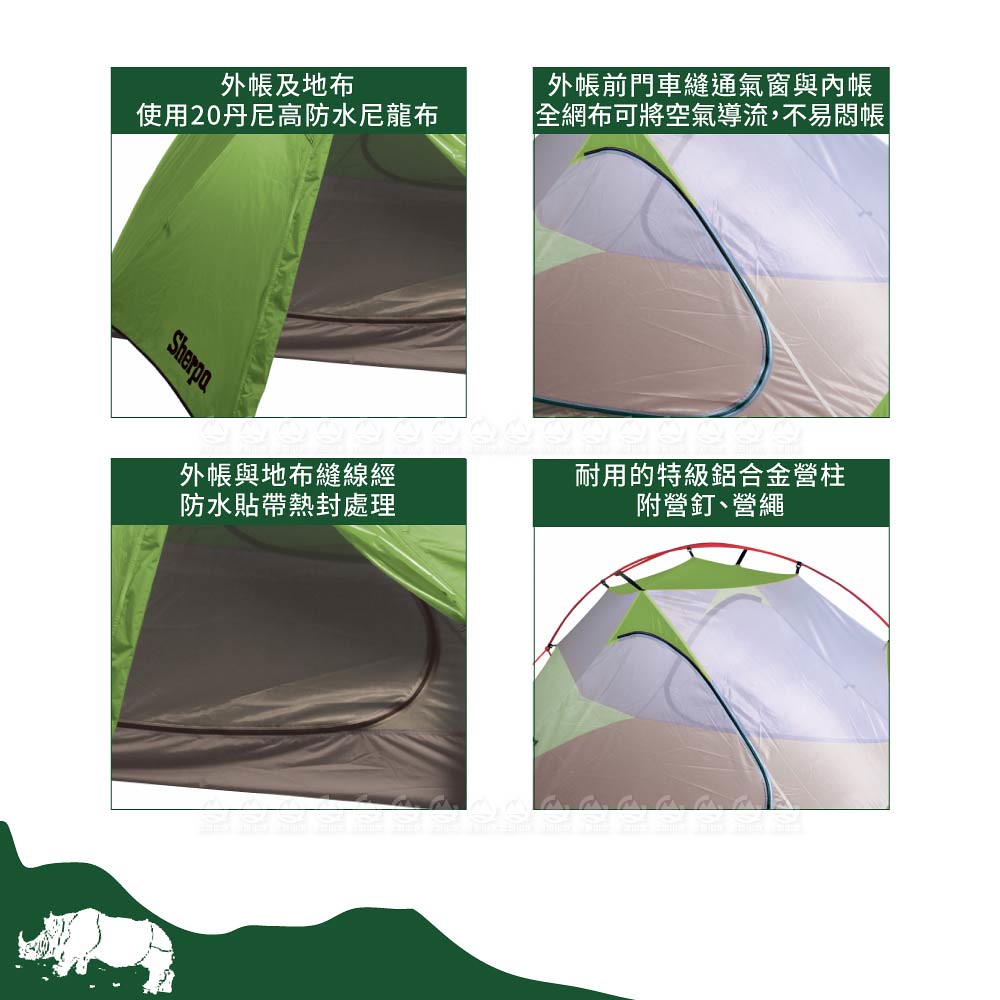The image features a digitally generated product advertisement for a Sherpa makeshift portable tent, ideal for camping and hiking. The white background is divided into four square photos arranged in a two-by-two grid, each depicting various views of the tent with a green horizontal strip at the top containing text in what appears to be Chinese. The top-left photo shows the exterior of the green and gray tent, while the top-right photo captures the tent seen through its netted window, showcasing green and blue hues. The bottom-left photo provides a glimpse of the dark gray, empty interior framed by green door flaps, and the bottom-right shows the tent's exterior again, emphasizing its green and blue color scheme. A distinctive green silhouette of a mountain with a white rhinoceros logo is located at the bottom left of the entire image.